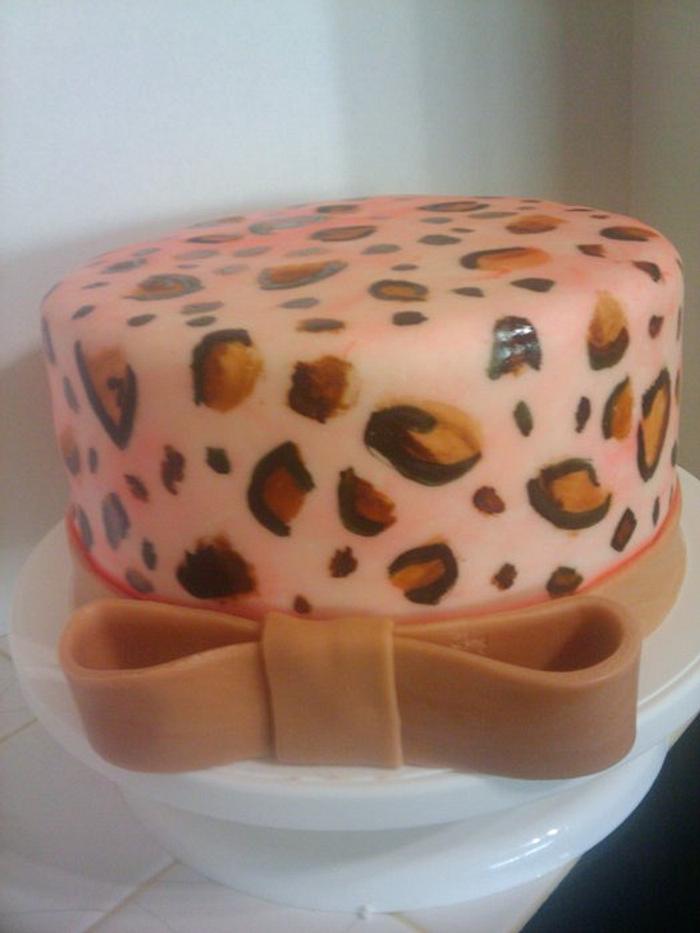This vertical rectangular image depicts an object that appears to be a decorative cake, though it could also resemble a hat or a bowl. The cake has a flat top and is predominantly salmon pink in color, adorned with a pattern of light brown spots outlined in dark brown, giving it an animal print appearance. A caramel-colored ribbon, resembling velvet, is tied around the bottom and sits on a white stand, which looks thick and plastic-like. The stand rests on what seems to be a white tile floor, and the background includes a plain white wall. Shadows are cast behind the stand, adding depth to the setting. The overall look is intricate and somewhat whimsical, with a definite sense of being a crafted decorative piece.